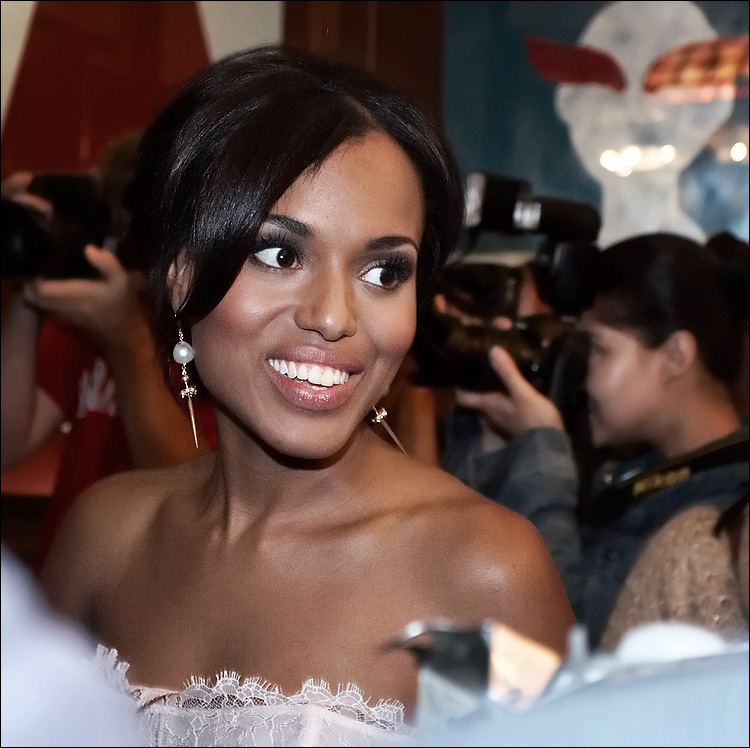In this image, we see an elegantly dressed African-American woman with long dark black hair, smiling and revealing her white teeth. She is positioned almost directly in the center of the frame, looking slightly to the right. Her attire includes a glimpse of a white lacy dress, long pearl earrings with gold accents hanging from the pearls.

The setting appears to be indoors, possibly during a formal or red carpet event, suggested by the presence of several photographers in the background holding large cameras. Despite the background being blurred, it's possible to discern some artwork on the walls. The colors in the image include light blue, white, brown, silver, gray, maroon, red, and dark blue. There is no visible text within the image.